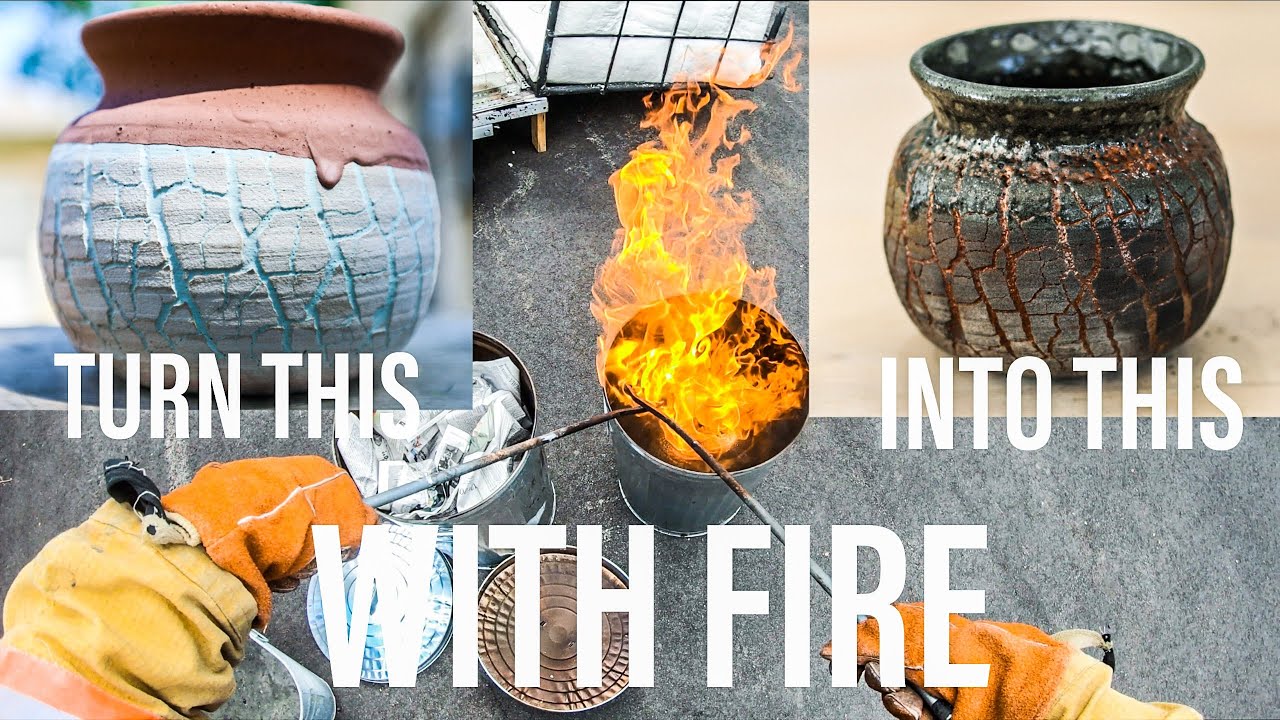The image depicts a detailed scene with a main photo and two smaller photos overlaid on the top left and top right corners. The central image shows a person, dressed in a heavy-duty yellow jacket and orange protective gloves, holding metallic prongs over a silver trash can that has flames coming out of it, all set against a gray asphalt floor. In the upper left corner, there is a photo of a raw, simple clay pot that is painted blue at the bottom and red at the top. This pot appears unfinished and rustic. Below this photo, there is text that reads "turn this." In the upper right corner, another photo shows a fully green, worked-on clay pot that appears finished and polished. This image includes the text "into this." Superimposed on the main photo are the words "with fire," indicating the transformative process. Together, the scene illustrates the use of fire to turn raw, unfinished pottery into a refined, completed piece.